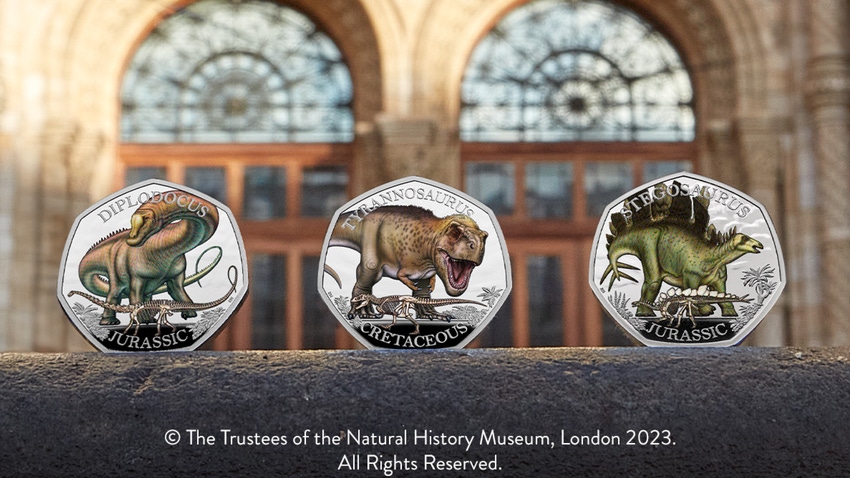In this detailed image taken at the Natural History Museum in London, three hexagonal silver tokens are prominently displayed on a stone ledge. Below them, small white text reads, "The Trustees of the Natural History Museum, London, 2023. All rights reserved." Each token features a different dinosaur and is labeled accordingly: the left token depicts a Diplodocus, labeled "Diplodocus" at the top and "Jurassic" at the bottom; the middle token features a Tyrannosaurus, with "Tyrannosaurus" on top and "Cretaceous" at the bottom; and the right token shows a Stegosaurus, labeled with "Stegosaurus" on top and "Jurassic" at the bottom. The tokens are placed vertically, allowing us to view them from the front. The background, slightly blurred, reveals the museum's historic architecture, including two large archways with glass panes set in wood frames, resembling church windows.